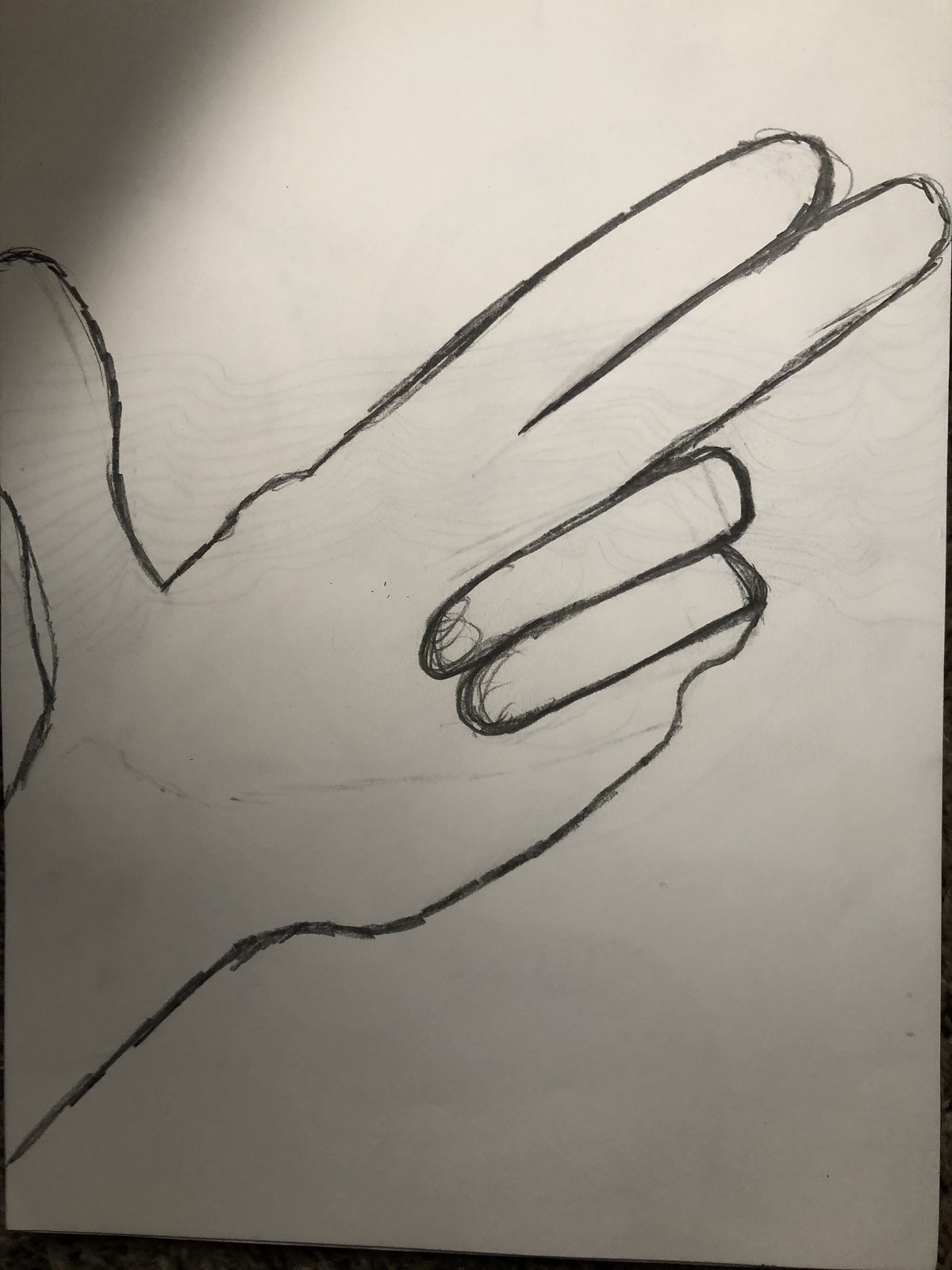A photograph captures a pencil or pen sketch on a white piece of paper, displaying an outline of a right hand. The hand appears to have been traced directly onto the paper, with its thumb pointing up, the index and middle fingers extended, and the ring and pinky fingers curled inward, forming the shape of a gun. The lines are sketchy and imperfect, with noticeable waviness and some tracing errors where secondary lines deviate slightly from the initial outline. Shadows are visible in the upper left corner of the paper, and faint wavy lines appear underneath the main sketch, possibly from another page behind or the back of the paper. The image is entirely black and white, devoid of any other colors.